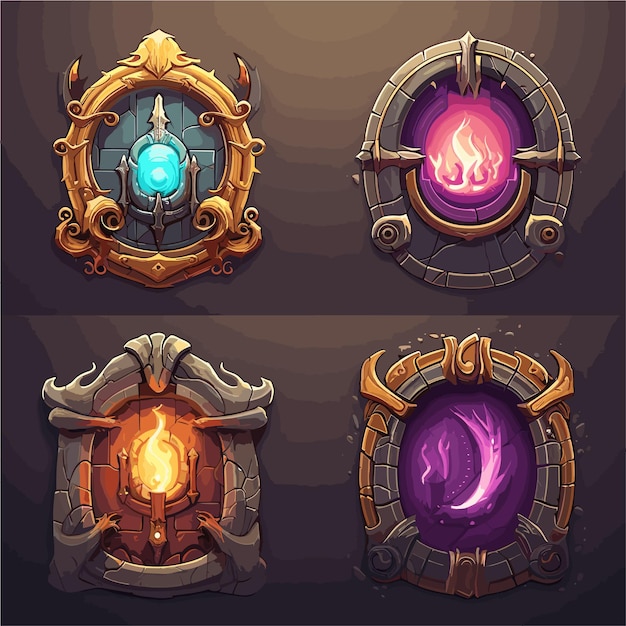The image features four digitally painted, fantastical objects or windows, each adorned with a distinct glowing element, set in ornate, oval frames with a medieval or video game aesthetic. Arranged in pairs with two on top and two on the bottom, these objects vary in color and material, and each emits a radiant glow that illuminates the intricate frames surrounding them.

- **Top Left**: This frame is embellished in gold and features a teal blue gem at its center, flanked by horn-like structures and other decorative motifs.
- **Top Right**: Encased in a stony grey frame, this window showcases a pinkish, fire-like element. The design includes textural details and circumferential patterns that suggest a glowing fire.
- **Bottom Left**: More irregularly shaped with a stony grey outline, this frame contains an orange, fiery center. The design incorporates arm-like extensions reaching from the frame toward the center, which emits a vivid glow.
- **Bottom Right**: This frame, outlined in a mix of gold and stony grey, features a purple, crescent-shaped swirl at its core that gives off an ethereal light. The perimeter is adorned with intersecting elements, enhancing its ornate appearance.

Together, these windows evoke a magical, medieval ambiance, reminiscent of elements one might find in a fantasy video game like Hearthstone.